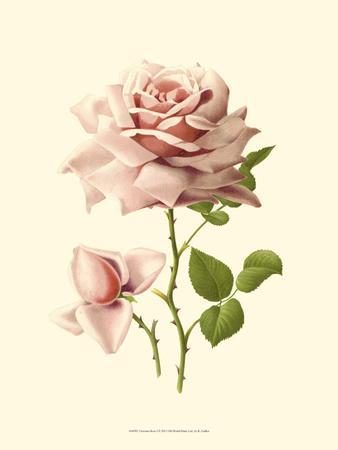The image features a detailed painting of two pink roses set against a cream-colored background. The larger rose is fully bloomed, with lush petals that dominate the composition. The green stem supporting the rose is adorned with sharp thorns and sprouting branches of verdant leaves. To the left of the main flower, a smaller rosebud is in the process of blooming, with three petals beginning to unfurl while the center remains closed. At the bottom of the image, a small line of text is visible but not legible. This elegant flower painting would be suitable for wall art or clip art.